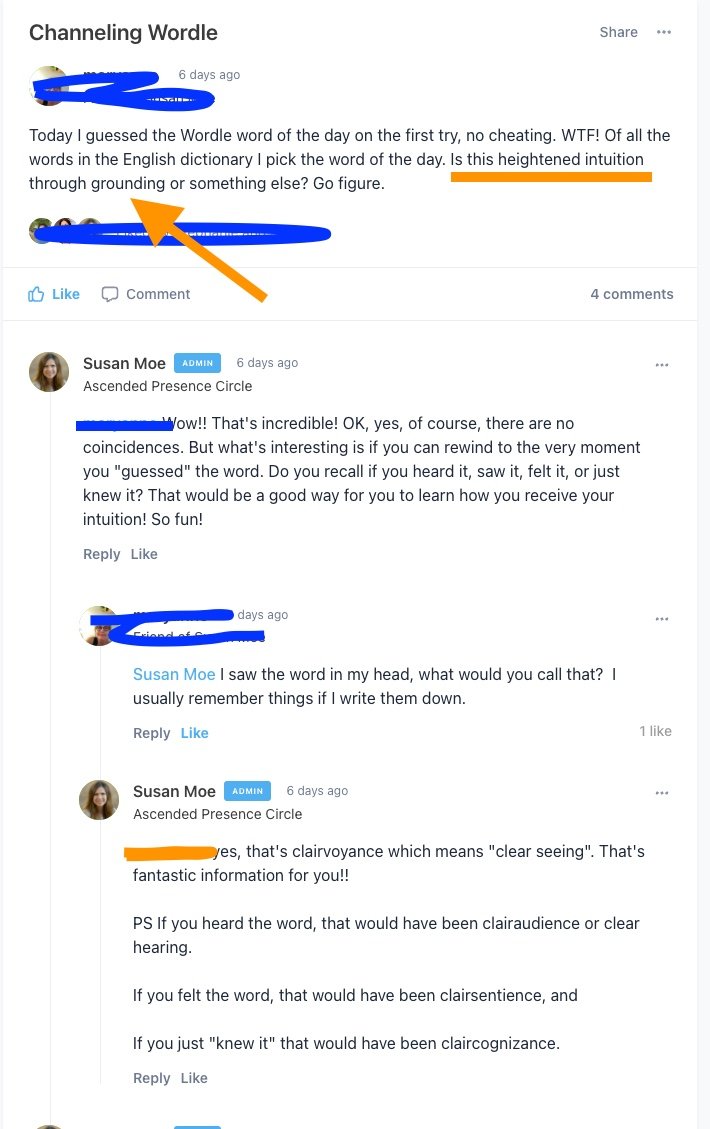This image appears to be a screenshot of a phone displaying a social media or messaging app interface. In the top left corner, the text reads "Channeling World," while in the top right, there is a "Share" option and a menu represented by three dots. 

The image has several sections obscured, primarily using a blue highlighter. The first paragraph and associated profile picture are completely crossed out in blue. Below this section are three additional profile pictures, also scratched out with the same blue highlighter.

There is an orange arrow superimposed on the image, pointing upwards toward the first obscured profile picture. Below the scratched-out content, a sentence partially underlined and highlighted in orange reads, "Is this heightened intuition?"

The second paragraph appears to be a response, presumably from a user named Susan Mo. This paragraph is dated six days ago and identifies Susan as an admin, indicated by the text "Ascendant Presence Circle." The person Susan is responding to has their identity colored out in blue. Susan's response includes a lengthy paragraph, in which several words are marked out in orange highlighter.